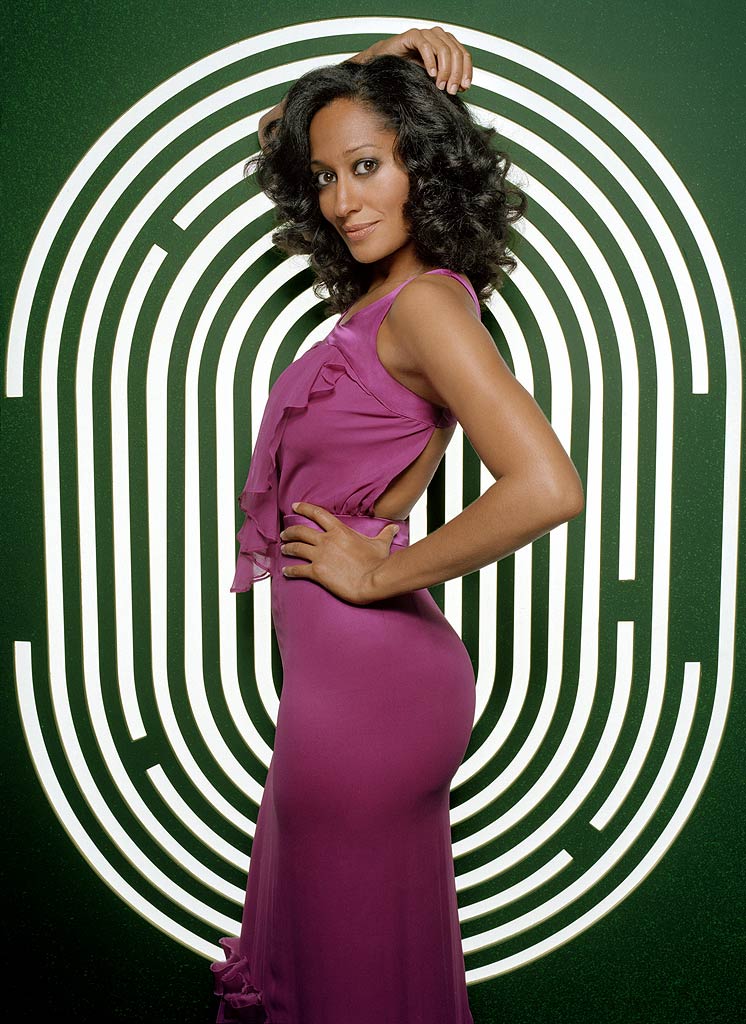This image captures Tracee Ellis Ross, daughter of Diana Ross, standing in a stylish and confident pose. She displays her natural dark curly hair cascading down, and she dons a mauve dress with ruffles along the neckline. The dress, with its pinkish and purple hues, exposes her back and gracefully drapes around her form. Tracee stands sideways, offering a side profile where her left arm rests on her hip, while her right arm is elegantly placed atop her head. Her makeup is applied subtly, complementing her glowing tan complexion, and she gazes into the camera with a soft smile or a smirk. The backdrop is green, featuring a large white oval shape, intricately designed with lines resembling a maze or fingerprint. This background highlights Tracee’s poised and radiant presence.